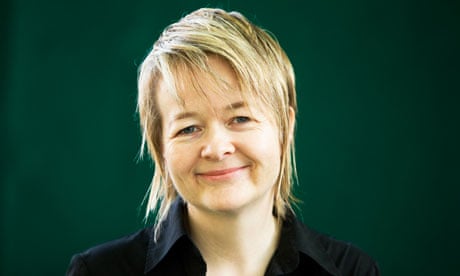This horizontally oriented photograph features a middle-aged woman with fair skin and light blue eyes, smiling gently at the camera. Her bleach blonde hair, which is shoulder length, is styled straight with some bangs and is swept to the right side of the image, partially framing her face. She is wearing light pink lipstick that complements her smile, revealing dimples on her cheeks. The woman is dressed in a black button-up shirt with an unbuttoned collar, though the image is cropped just below her neck, providing limited detail about her attire. The background is a solid, almost emerald green, giving a professional appearance that suggests this could be a corporate headshot.